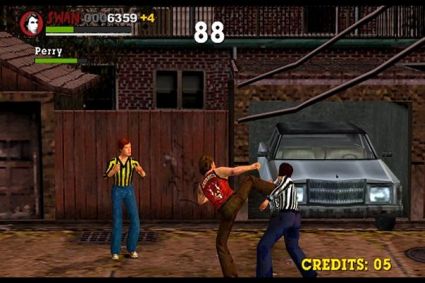This is a screenshot from an older-style side-scrolling or fighting video game set in a 70s-like environment. The scene depicts a physical confrontation involving three men, with two engaged in a fight and one standing ready to join. The man delivering a powerful kick is wearing a red tank top with brown pants, his right fist raised. The man being kicked is clad in a long-sleeved black and white striped shirt paired with dark blue jeans. A third individual, also in a striped shirt and jeans, stands nearby with fists up, ready to fight. The background features a gray or silver convertible car inside an open garage and a large brown house, indicative of a residential street setting. The top of the screen displays various game elements: the word "swan," a small circular image of a person with a mysterious sequence of numbers "0 0 0 6 3 5 9 +4" next to it, and a green health bar labeled "peri." Prominently centered at the top is the number "88" in white. In the lower right corner, the credits read "0-5" in yellow.